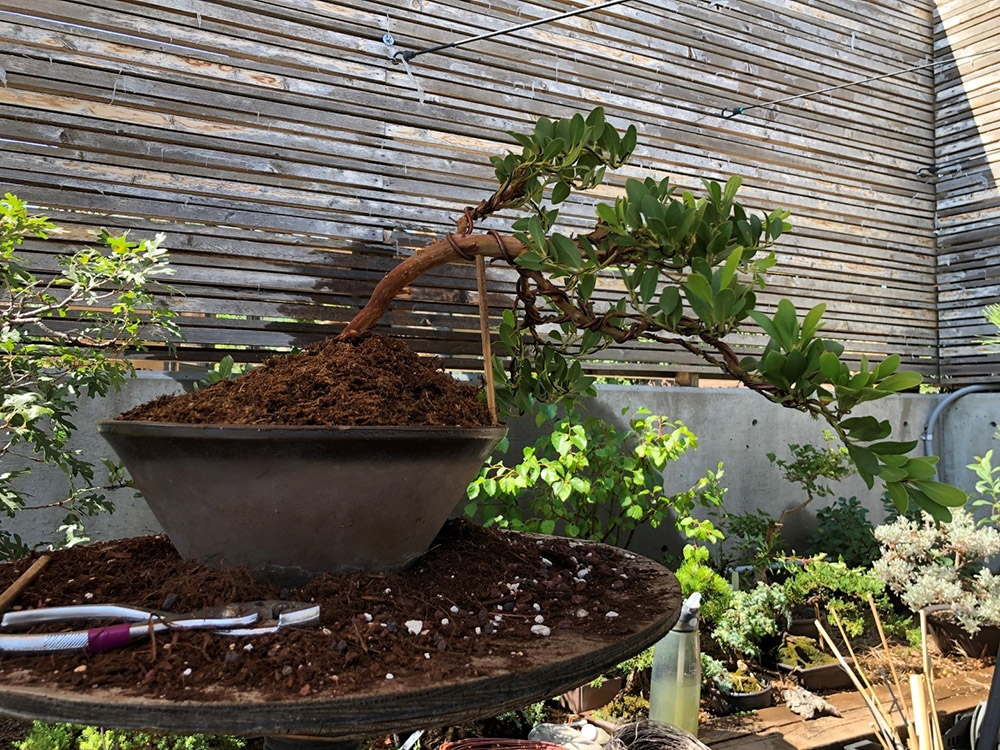The photograph depicts a serene indoor bonsai garden, evidently illuminated by sunlight. Central to the image is a rounded dark brown plant pot, possibly made of clay, perched on a circular wooden pedestal. The pot contains a mound of brown soil that slightly overflows its edges. From this soil, a miniature bonsai tree, characterized by its thin brown trunk and sprawling branches adorned with dark green leaves, leans prominently to the right.

Surrounding this focal point are several other plant pots, neatly arranged on benches made from wood. These pots house diverse plants, primarily displaying an array of lush green leaves, although one plant stands out with its unique white foliage. Scattered around the pots are essential gardening tools, including a pair of silver pliers and watering bottles, indicating active care and maintenance of the bonsai collection. The backdrop consists of horizontal gray wooden boards forming a fence that extends upwards, positioned above a sturdy gray concrete wall. Sunlight filters into the garden, enhancing the tranquil and meticulously curated space.